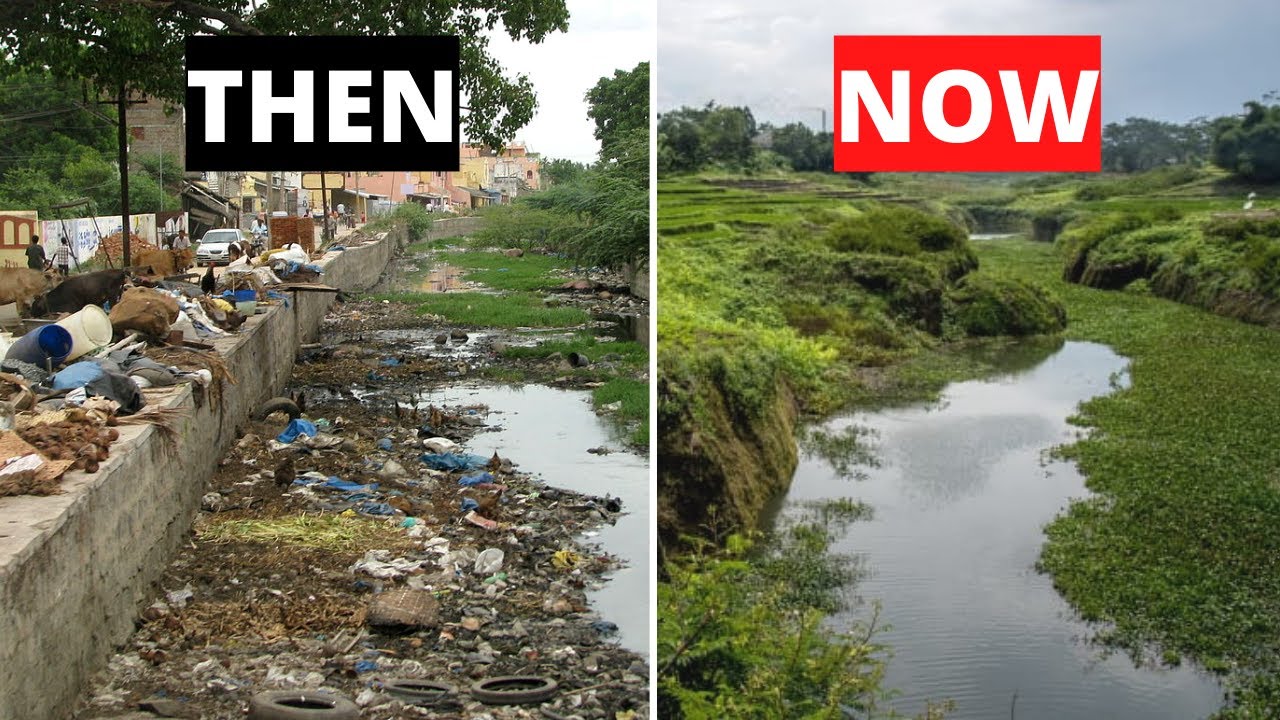This image shows a striking before-and-after comparison of a waterway, divided into two sections with a white border in landscape layout. On the left side, marked "THEN" with black text on a black bar, the waterway is filled with various types of trash, including tires, plastic bottles, tarps, and plastic barrels. The concrete bank and nearby area are also littered with debris, and some distant buildings in creams and pinks can be seen in the background. Additionally, there are a few people walking around the polluted area. In contrast, the right side, labeled "NOW" in white text on a red bar, depicts a transformed scene with a clear pond, lush greenery, and a blue sky. The once-trash-filled area is now pristine, free of all visible garbage, people, and buildings that were previously shown in the "THEN" image. This cleaned-up version offers a serene and revitalized landscape.